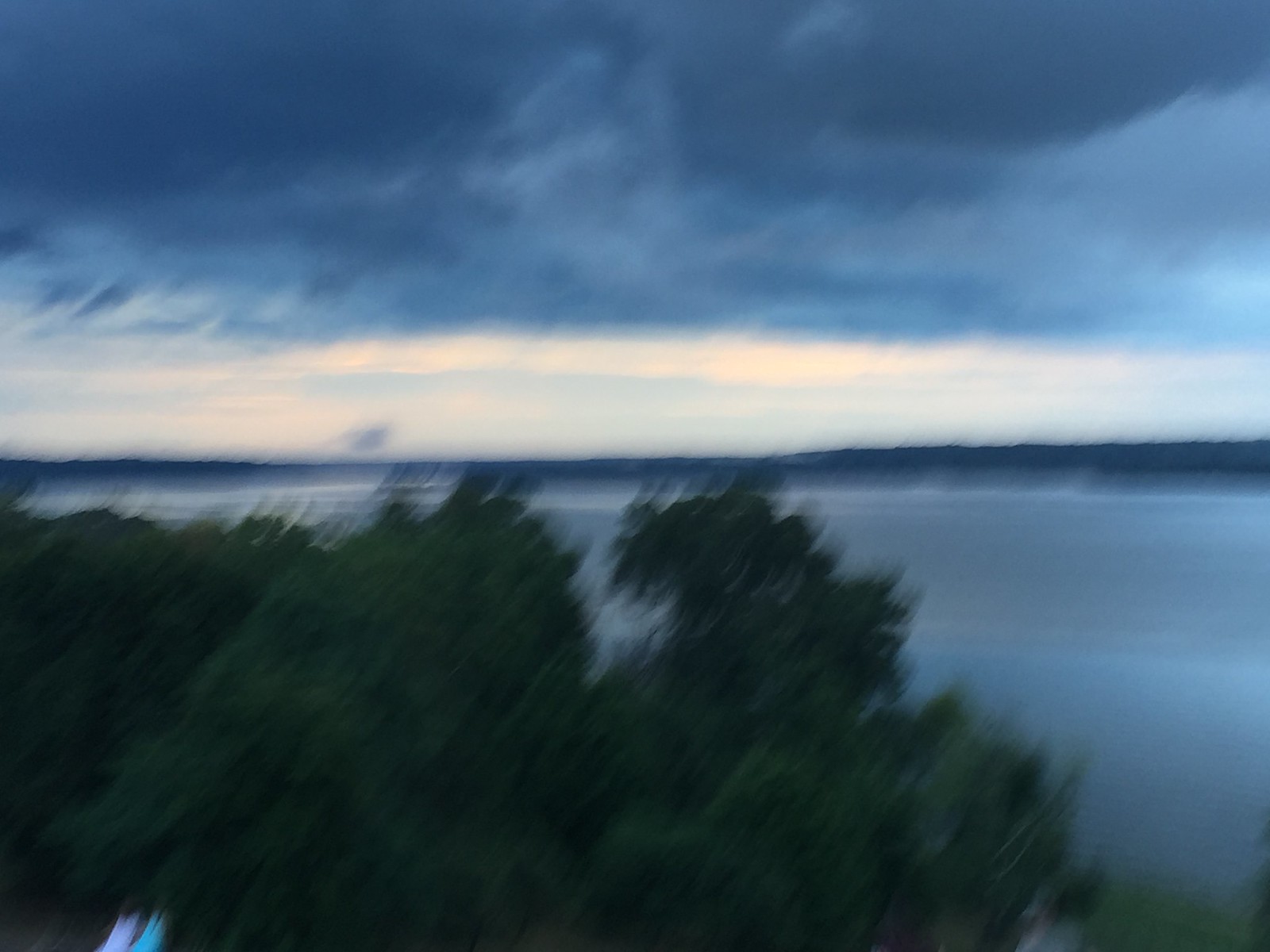This blurry and unfocused photograph captures an outdoor scene featuring a lake surrounded by trees and bushes. The image appears as though it was taken with the camera in motion, resulting in a very fuzzy appearance. The lake's water spans from the bottom foreground to a distant horizon, creating a light blue expanse that darkens toward the far shore, hinting at dusk or evening light. On the horizon, a band of trees frames the scene, with additional trees and bushes appearing closer to the camera. The sky above shows a mix of dark, almost stormy clouds at the top, transitioning into lighter clouds and patches of blue sky closer to the horizon. In the bottom left corner, two indistinct figures stand side by side, one in purple and the other in turquoise. The bottom right corner reveals a grassy area, adding texture to the foreground of this otherwise blurred landscape.